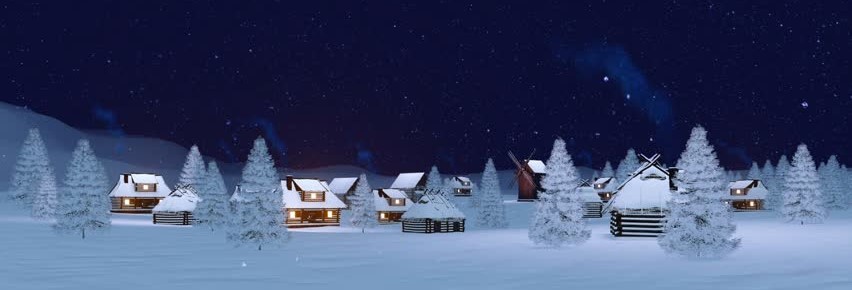The image is a digital painting of a serene, snowy village nestled in a wintery, wooded area under a starlit navy blue night sky. The scene showcases a collection of small log cabins with warm, inviting lights glowing from the windows, positioned in the center, behind a foreground of snow-covered pine trees. The cabins are randomly arranged, creating a quaint town vibe. The ground, trees, and cabins are all blanketed in pristine white snow. wisps of smoke gently rise from the chimneys of the cabins, adding a sense of warmth to the cold night. In the background, snowy white mountains and hills stretch across the left side creating the horizon, while a dense grove of tall, snow-covered pine trees forms the horizon on the right. The sky above is dotted with countless stars, enhancing the tranquil, magical atmosphere of this winter night scene.